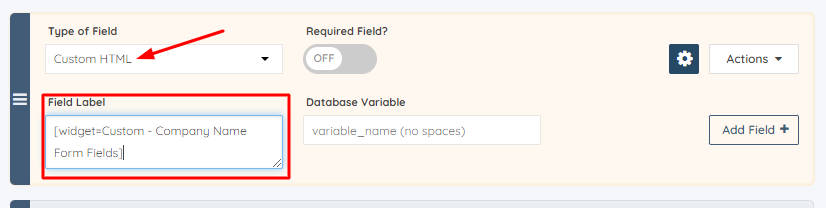The image is a long rectangular layout with a cream-colored background. On the left side, there is a slim, dark blue border featuring three white horizontal lines in the middle. 

In the central area of the image, towards the top left, there is a field with a drop-down bar labeled "Custom HTML," highlighted by a red arrow pointing to the HTML text. Adjacent to this field is a toggle switch labeled "Required Field?" 

To the far right of this toggle is a gear icon, representing a settings button, which likely offers additional drop-down actions.

Further down in the image, there's a section marked "Field Label." Within this section, text is entered in brackets as "[widget=custom-company name form fields]," and this text is emphasized with a red box drawn around it.

To the right of this is a label "Database Variable," accompanied by an input field labeled "variable_name" with a note in parentheses advising "no spaces."

On the far right side of the image, there is an "Add Field +" button.

At the bottom, a long, slender bar is partially filled with a black color, providing a subtle visual separator.